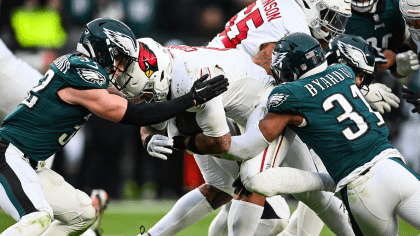This photograph captures a dynamic moment during an American football game between the Philadelphia Eagles and the Arizona Cardinals. At the center of the frame, a Cardinals player wearing a white jersey and a white helmet, which features a distinct red cardinal logo, is seen attempting to run the ball. He is being tackled by two Eagles players. The Eagle on the left is clad in a dark green uniform with a green helmet adorned with white eagle wings. This player is wearing black gloves and the white coverings on their forearms are visible as they wrap their arms around the Cardinal. Another Eagles player, similarly dressed with white sleeves, is also engaged in the tackle, gripping the Cardinal player's legs. In the backdrop, the blurred figures of additional players from both teams and indistinct spectators highlight the intensity of the game on the vibrant green field.